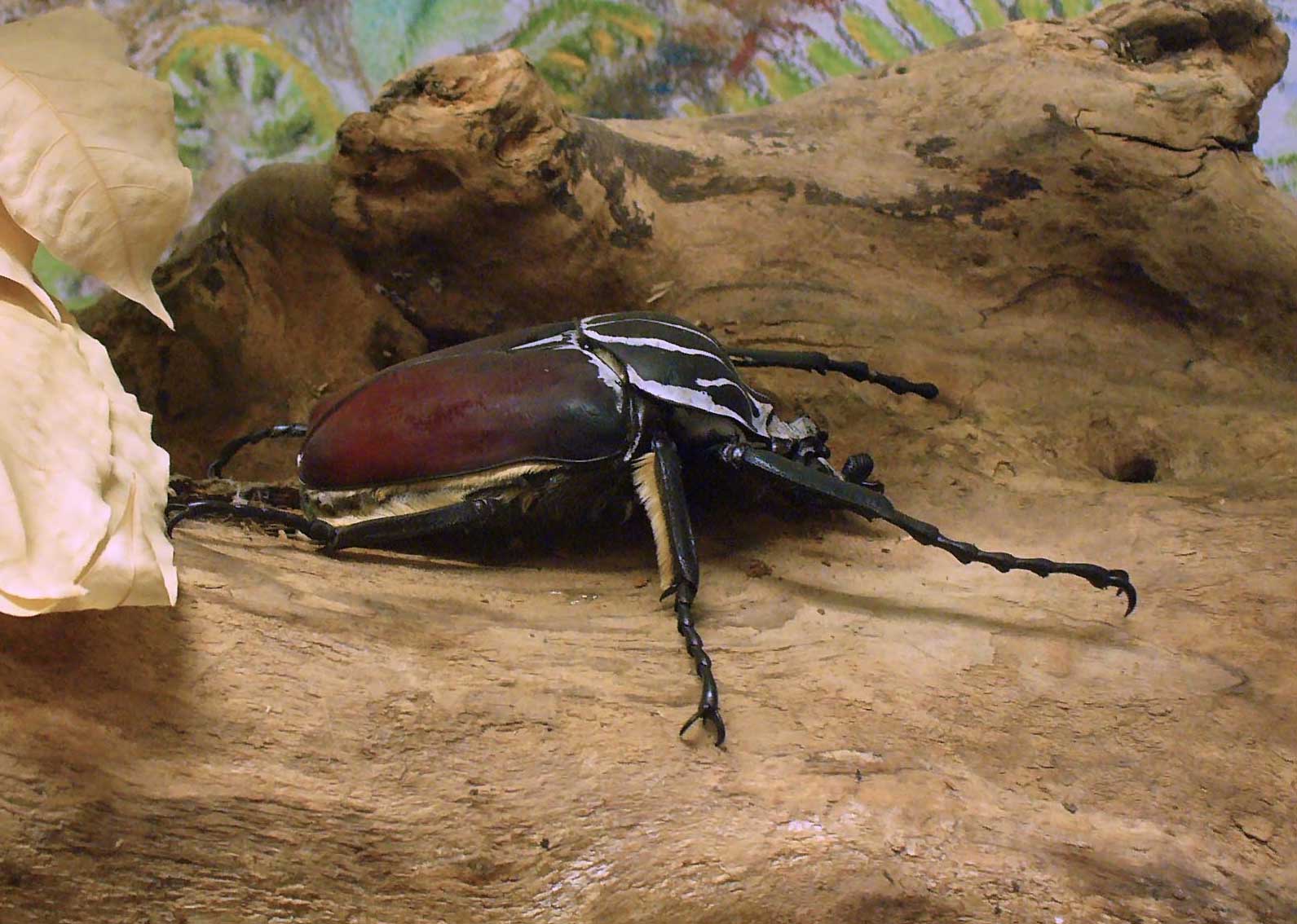This highly detailed, close-up image showcases a large beetle occupying the central portion of the frame. The beetle's body features a distinctive coloration: the torso is a rich burgundy red with black accents, while the head is black adorned with white and gray stripes. The beetle's six black, ridged limbs curve at the ends, resembling claws or claspers designed for gripping. Its legs extend outward, with some potentially feather-like structures near the second half, likely aiding in sensory perception. The creature's segmented wings lie flat against its torso, displaying a gradient from black at the top near the head to dark red towards the bottom.

The beetle sits atop a tan-colored surface, possibly an old tree stump or rock. This surface exhibits significant texture, especially behind the insect, suggesting an aged, weathered material. To the right of the beetle’s head, there's a noticeable hole, adding to the textured complexity of the background. To the left, some tan-colored leaves are visible, which might be artificial. The overall scene captures the intricate details of the beetle and its naturalistic setting vividly.